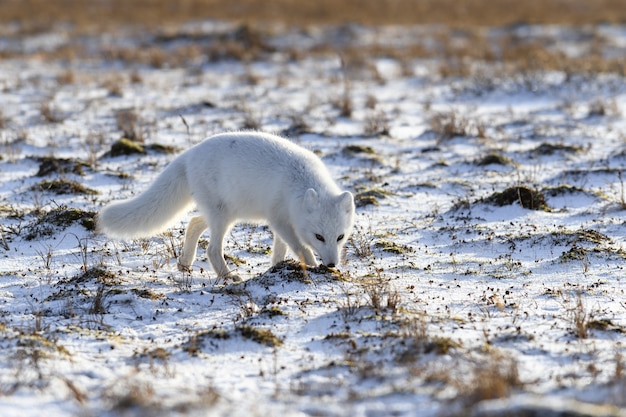In this captivating outdoor scene, an enchanting white fox stands out against the snow-dusted landscape. The sparse snow cover reveals patches of brown earth and sprigs of hardy vegetation, creating a varied backdrop that breaks the monotony of the wintry setting. The fox, with its plush, bushy tail and pristine white fur, gracefully navigates the field, its dark eyes and nose providing a striking contrast to its snowy coat. With its head lowered, it appears to be intently sniffing or possibly hunting, blending seamlessly into its surroundings with its perfect natural camouflage. The foreground highlights the fox and the immediate plants with sharp clarity, while the background softly fades into a blur, emphasizing the serene and chilly essence of this natural habitat.